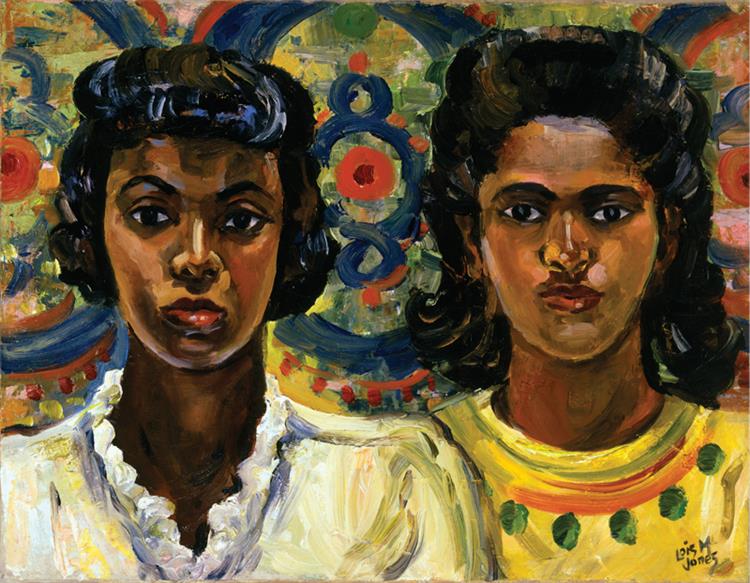This watercolor painting by Lois M. Jones portrays two African-American women standing side-by-side, likely set in the 1950s based on their attire and hairstyles. The woman on the left wears a white v-neck shirt with ruffled details, while the woman on the right dons a distinctive yellow blouse featuring green leaf-shaped ornaments and streaks of red at the collar. Both have dark hair and wear red lipstick, with one appearing slightly older and darker-skinned than the other. Their haircuts are relatively short. They stand against an extraordinarily bold and colorful background, which could be a store display or vibrant wallpaper, characterized by dominant hues of green, blue, pink, and traces of orange forming a circular pattern. The artist's signature, "Lois M. Jones," is located in the lower right corner, rendered in black paint.